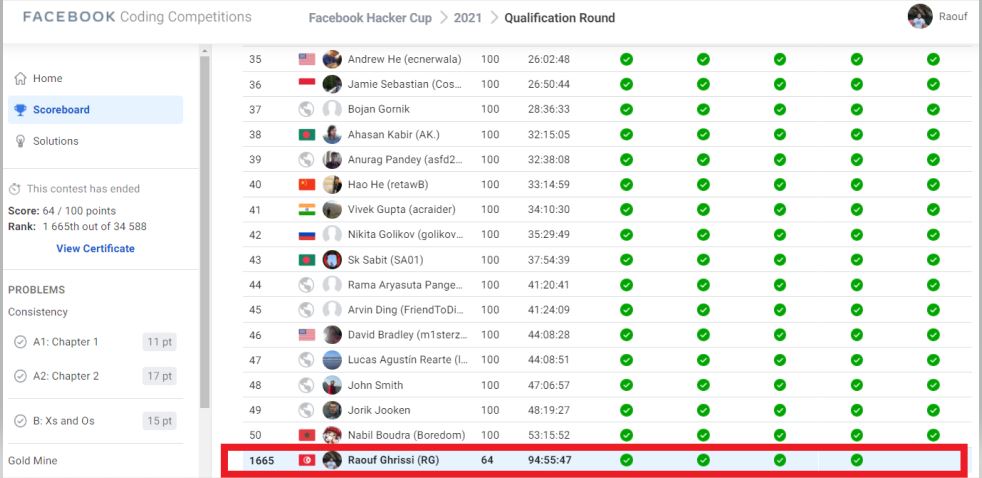This image is a screenshot taken from a webpage on Facebook, specifically showcasing the results of the Facebook Coding Competitions' Hacker Cup 2021 qualification round. The main focus is on a participant named Raul. Although his profile picture is displayed, it is too small to be clearly visible and is positioned on the left side of the vertical navigation menu. 

The highlighted section on the menu is the 'Scoreboard,' which is indicated by a blue highlight. Other available sections in the menu include 'Home' and 'Solutions.' The page clearly indicates that the contest has concluded. Raul's score is prominently displayed as 64 out of 100 points, and his rank is shown as 166 out of 34, although this might be a misprint and means 166 out of 3400 or another larger number.

A clickable blue link titled 'View Certificate' suggests that participants can obtain their completion certificates. Below this, there is a section detailing 'Problems Consistency' with some unspecified numerical data. Within a white box at the bottom, a problem named 'Gold Mine' is listed.

Further down, a detailed ranking list ranges from positions 35 to 50. This list includes participant names, some accompanied by profile pictures. Raul appears to be the top scorer with the ID 191665. His score is emphasized by his entry being outlined in a thick red marker, in contrast to the other participants who have five green dots next to their names.